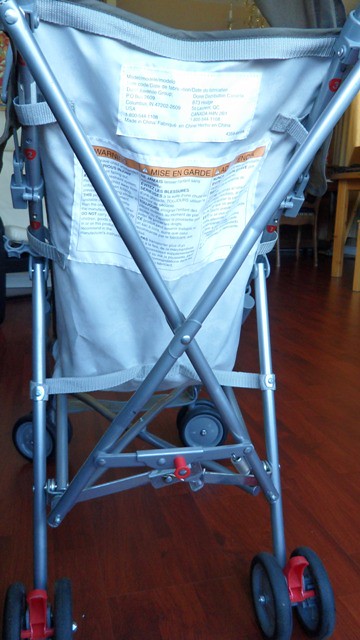This photograph captures the back view of a wheelchair-like device, possibly a hospital wheelchair or stroller, set against a dark, red-tinted wooden floor. Dominating the frame with its light blue metallic frame, the seat is constructed from a tough material, which might be plastic, cloth, or burlap. 

The back of the device features two noticeable white tags, possibly for safety information, with dark, unreadable printing due to light and distortion. Beneath these tags, there's a larger label featuring an orange strip at the top, followed by densely-packed black text, suggesting detailed instructions or information.

The wheelchair/stroller has a total of eight black rubber tires, with each wheel capable of a 360-degree spin. The wheels are supported by sturdy, crisscrossing metal beams. Additionally, there are red brakes and pins on the frame, hinting at functionality for folding and portability. Small details like button mechanisms on the poles further indicate ease of folding and carrying.

The setting appears indoors, with a suggestion of chairs placed nearby, but they are largely obscured by the prominent device in this highly detailed and focused capture.